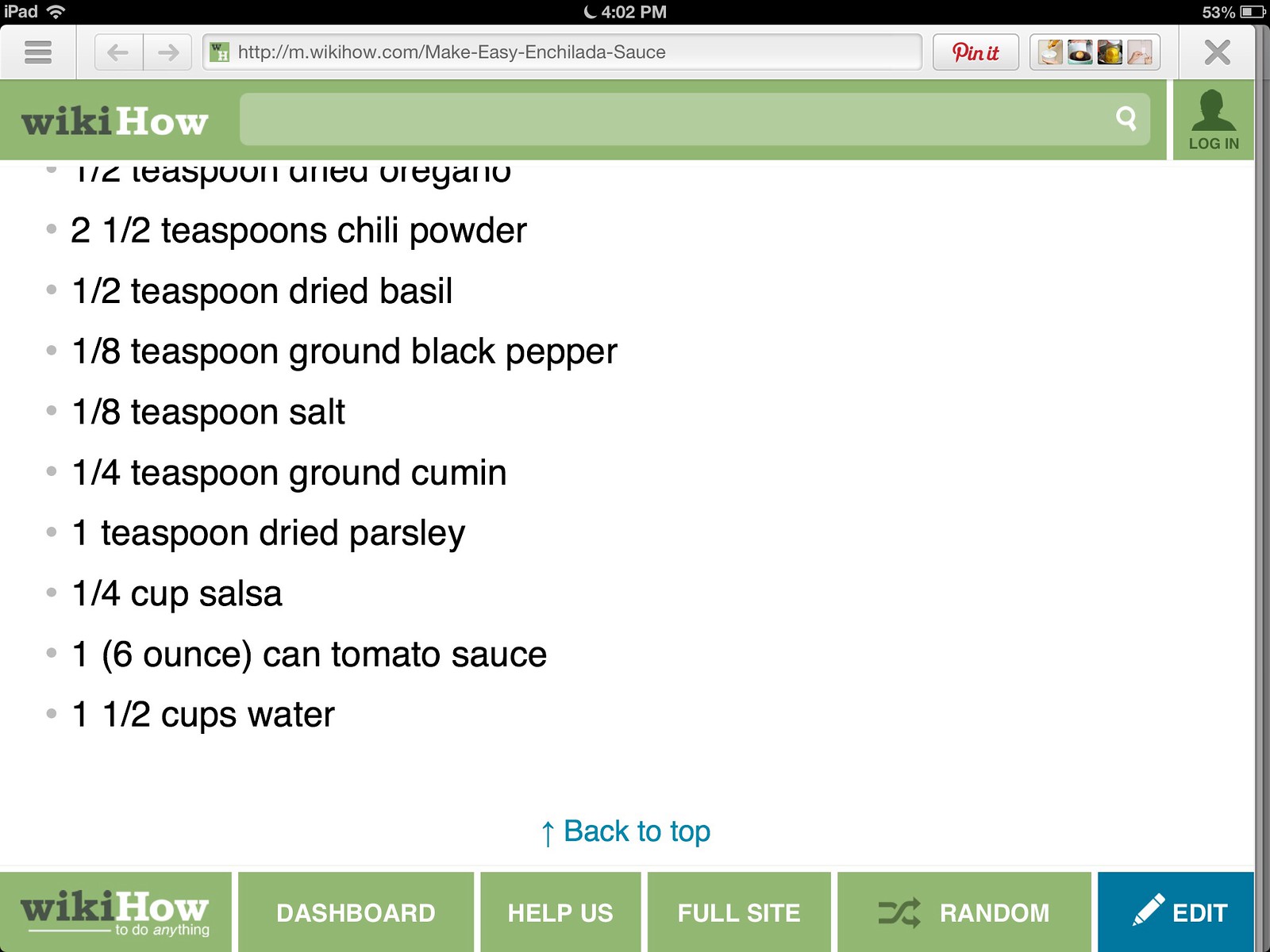The image is a detailed screenshot from an iPad, showcasing a web page on wikiHow. At the very top-left, the screen indicates "iPad" along with a Wi-Fi signal and the time 4:02 p.m. The top-right features a moon symbol and shows 53% battery power. Below this, the address bar displays the URL: http://m.wikihow.com/make-easy-enchilada-sauce. The wikiHow page itself has a green header with navigation options including "Pin it" and other symbols. Central to the screenshot is the main content area, showing a bullet-point list of ingredients for an enchilada sauce recipe: 1 1/2 teaspoons dried oregano, 2 1/2 teaspoons chili powder, 1/2 teaspoon dried basil, 1/8 teaspoon ground black pepper, 1/8 teaspoon salt, 1/4 teaspoon ground cumin, 1 teaspoon dried parsley, 1/4 cup salsa, 1 6-ounce can of tomato sauce, and 1 1/2 cups of water. Towards the bottom of the page, there's a "Back to top" link in blue, and at the very bottom, another green banner with options such as "wikiHow to do anything," "dashboard," "help us," "full site," "random," and an "edit" button in a blue square.